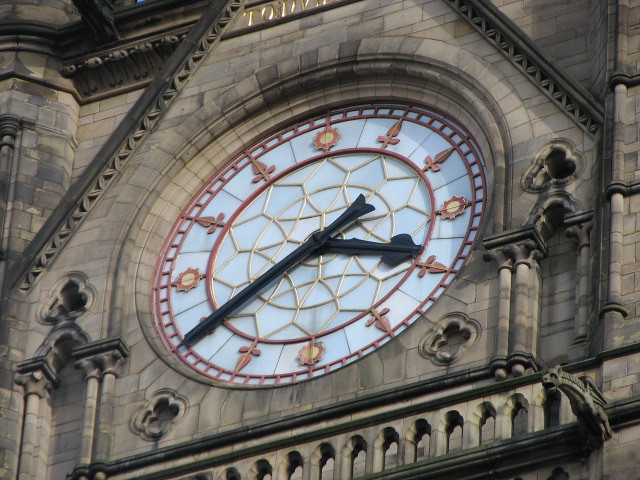A detailed photograph showcases an ornate clock mounted on the exterior of a church. The clock features a striking blue stained glass face, devoid of numerical markings, instead displaying small, intricate objects indicating the hours. Surrounding the clock's face is a robust frame of brown bricks, embellished with carved club patterns. The clock's black hands indicate the time as 3:40. Adding to the gothic charm, a pair of gargoyles are positioned on either side of the clock, further enhancing the architectural detail and historical ambiance of the scene.